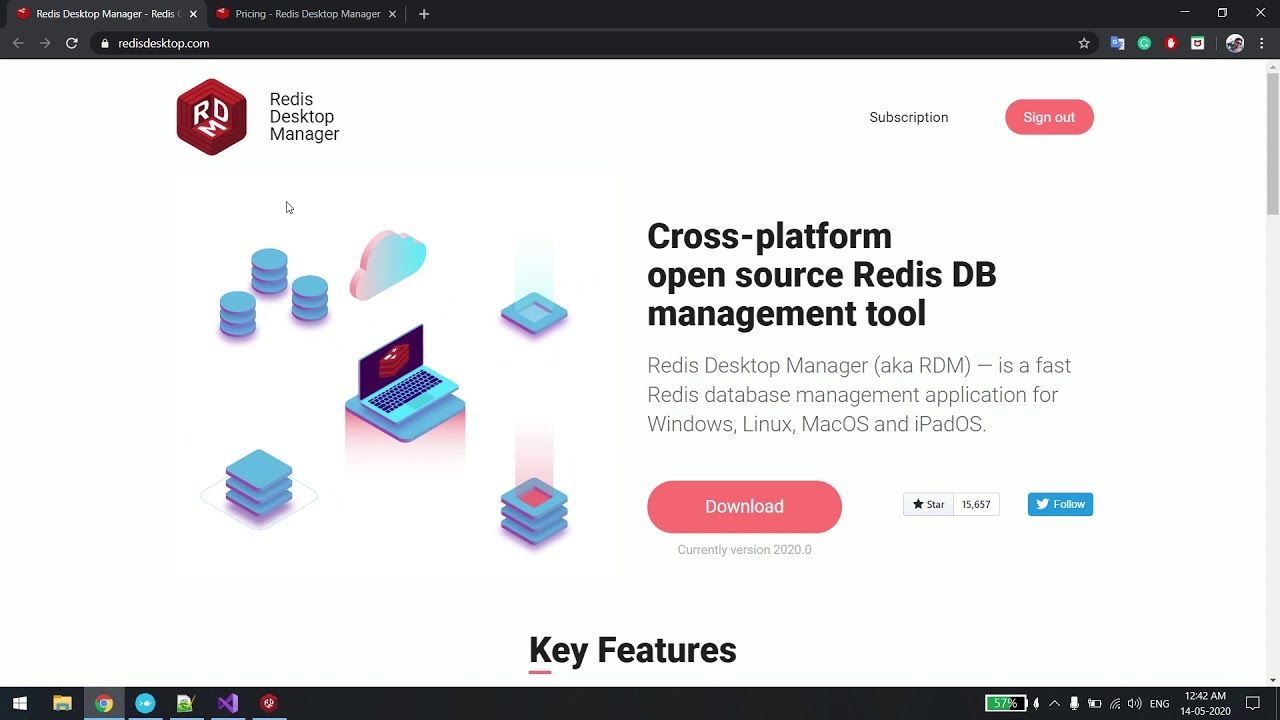This image is a detailed screenshot of a web browser window displayed on a Windows desktop. The browser has two tabs open, with the active tab displaying the website redisdesktop.com. The selected webpage is the landing screen for Redis Desktop Manager, an open-source, cross-platform database management tool specifically for Redis. 

The webpage prominently features IT-related graphics on the left side, including illustrations of laptops and clouds, indicating its connection to technological applications. On the right side, the text clearly states the name of the tool and its purpose. Below this information is a prominent red button offering an option to download the current version of the software, labeled 2020.0. 

Additionally, the top of the screen includes navigational buttons for "Subscription" and a red "Sign Out" button. The screenshot also captures the Windows taskbar at the bottom, where various desktop icons are visible, including shortcuts to applications, the battery status, system time, and other standard desktop indicators.